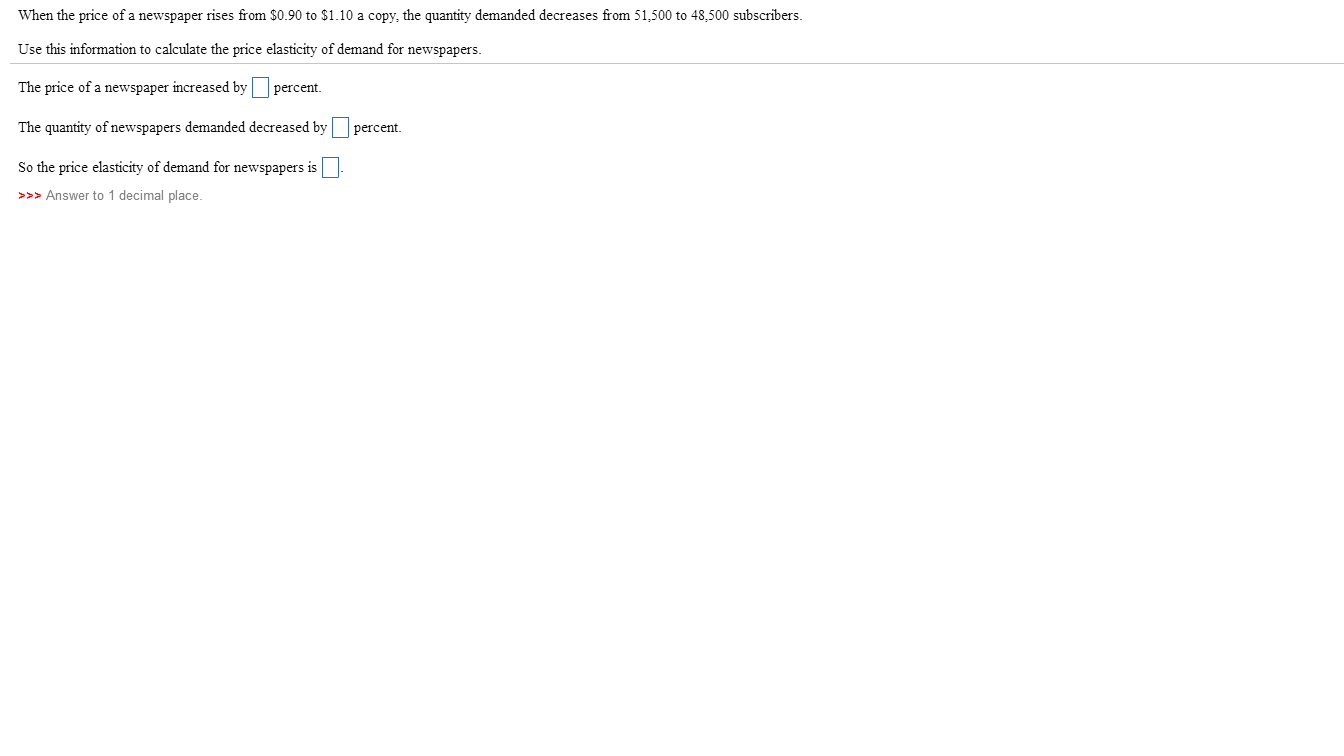This image depicts a web page with a plain white background and six distinct lines of text in black. The text provides an example calculation for the price elasticity of demand for newspapers. 

1. The first line reads: "When the price of a newspaper rises from $0.90 to $1.10 a copy, the quantity demanded decreases from 51,500 to 48,500 subscribers."

2. The second line instructs: "Use this information to calculate the price elasticity of demand for newspapers."

3. The third line presents: "The price of a newspaper is increased by [blank]%." 

4. The fourth line states: "The quantity of newspapers demanded decreased by [blank]%."

5. The fifth line concludes: "So the price elasticity of demand for newspapers is [blank]."

The final sixth line includes three red arrows pointing to the right, followed by the instruction in gray font: "Answer to one decimal place." Each blank space designed for answers is represented as a square box with a blue outline. The overall layout is straightforward, with all instructional text in black and the additional directive in gray, maintaining a clear and easy-to-follow format.